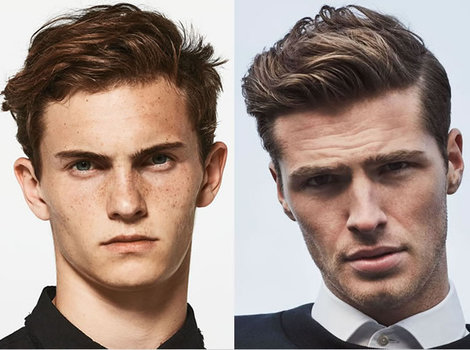This is a detailed side-by-side photo of two Caucasian men standing in front of a white background. On the left is a younger man, likely around 19-20 years old. He has short, tussled dark brown hair, thin brown eyebrows, and blue eyes. His face is covered in freckles, and he has thin lips with a serious, almost upset expression. He is wearing a black collared shirt. On the right is an older gentleman, perhaps around 30 years old, with blondish-brown hair that is longer on the top than on the sides, styled in a modern fashion. His eyes are obscured by a shadow, but he has full pink lips and a slightly scruffy beard that appears to be about 2 or 3 days old. He is dressed in a white button-up shirt with the top button fastened and a black sweater over it. His small ears add to his distinctive look. Both men have a serious demeanor, captured in a well-lit, realistic photograph.